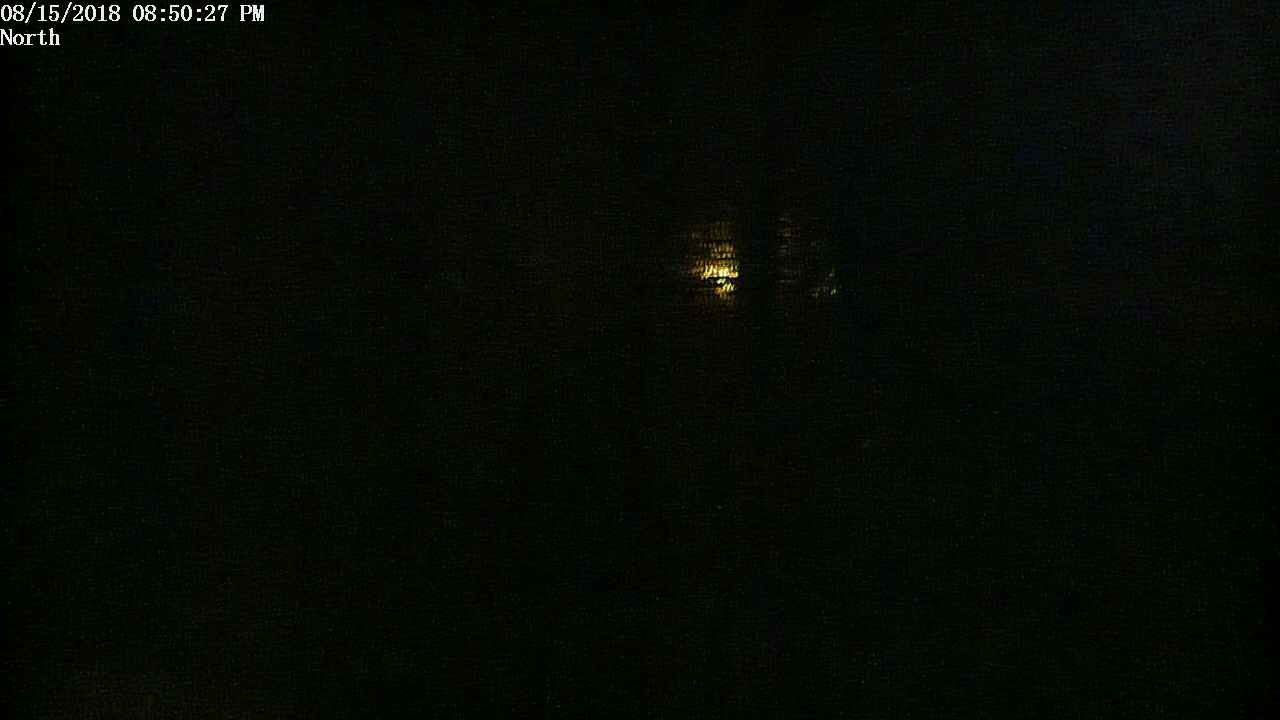In this dark photograph, predominantly black with minimal visible details, a distinct yellowish-green light emanates from what appears to be a cabin or shack situated more towards the right-center of the image. This light is partially obscured by the silhouettes of nearby trees or possible barriers, creating a haunting scene. The light source seems divided, with the left side appearing brighter than the right. In the top left-hand corner, white text marks the date "08-15-2018" and the time "08:50:27 PM," along with the direction "North," providing a precise timestamp and orientation for the photograph.